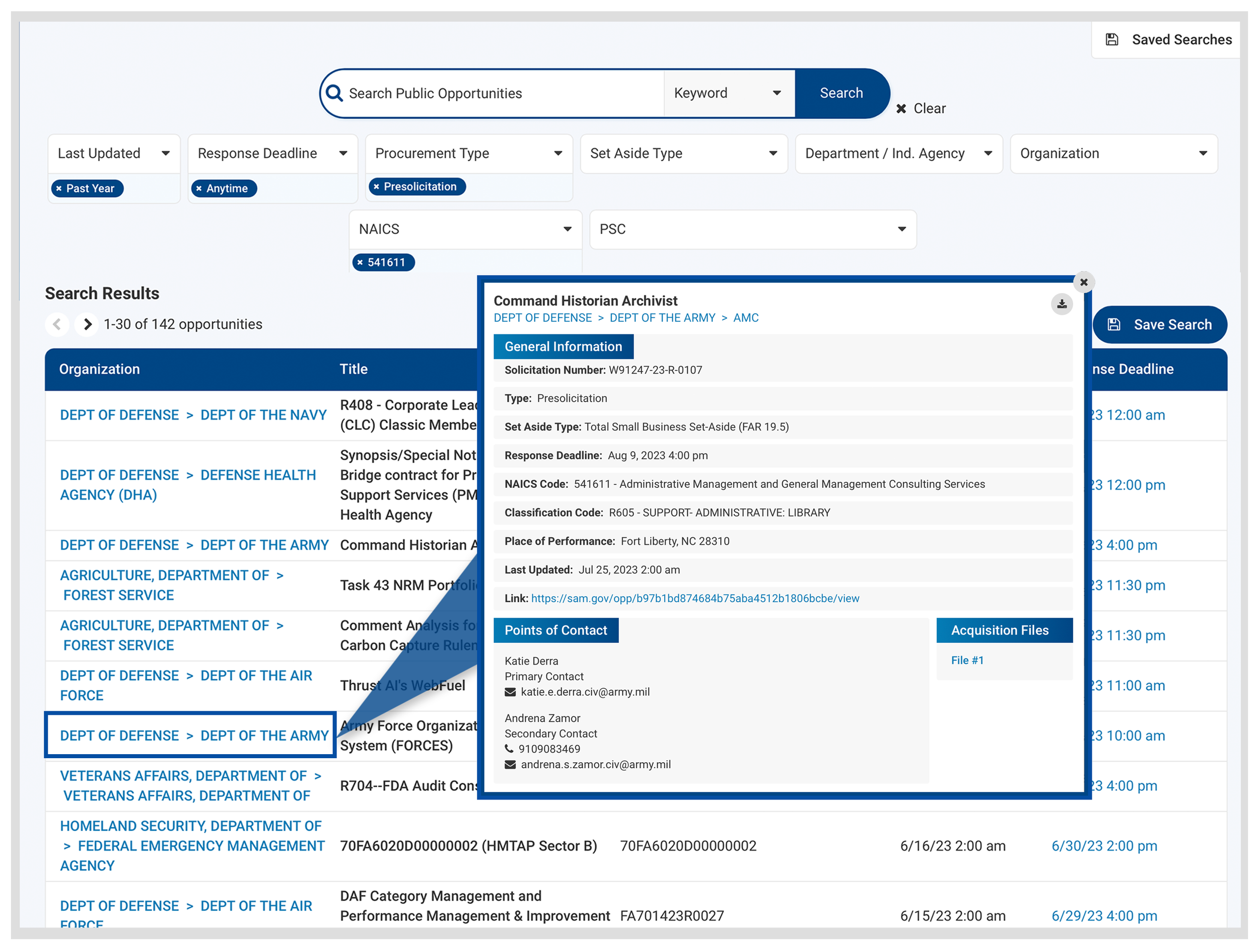The image is a detailed screenshot of a public database website designed for searching various opportunities. At the very top, there is a search bar labeled 'Search Public Opportunities,' which includes a keyword drop-down menu and a dark blue 'Search' button. Below this, users can refine their search with multiple criteria such as 'Last Updated,' 'Response Deadline,' 'Procurement Type,' 'Set-Aside Type,' 'Department or Industry Agency,' 'Organization,' 'NAICS,' and 'PSC.'

In the search results section, it displays entries 1 through 30 out of 142 opportunities. The organizations listed include the Department of Defense (with various branches like the Navy, Defense Health Agency, Army, and Air Force), the Department of Agriculture (specifically the Forest Service), Veteran Affairs, and the Department of Homeland Security.

A specific search result is surrounded by a dark blue box highlighting an opportunity from the Department of Defense, Department of the Army. A pop-up box provides more detailed information about this specific job listing for a 'Command Historian Archivist.' It includes the solicitation number, type, response deadline, and points of contact, showcasing various names for further communication.